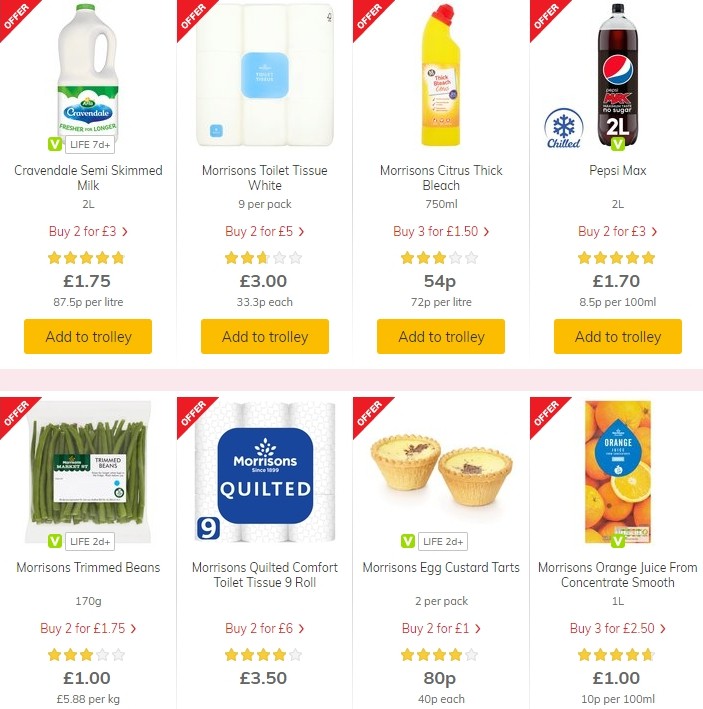The image caption appears to describe various grocery items along with their quantities, prices, and ratings. Here is a cleaned-up and detailed version:

"Displayed are a variety of grocery items available for purchase:

- **Item 1**: Unknown item at 5 grams for 3 pounds, rated 5 stars. Priced at 1.7 pounds with a conversion rate of 7.5 pounds per liter. 
- **Trolley Tissue**: 9-pack available for an additional offer.
- **Item 2**: Another variant at 5 grams for 5 pounds, available in different weights of 2.5 pounds, 3 pounds, and 3.3 pounds each.
- **Citrus Thick Bleach**: 750ml bottle, priced at 5 grams for 1.5 pounds, rated 3 stars. Priced at 54 pence, with a rate of 72 pence per liter.
- **Pepsi Max**: 102 liters offered at 5 grams for 3 pounds, rated 5 stars and weighs 1.7 pounds. The conversion rate is 8.5 pounds per 100ml.
- **Trimmed Green Beans**: Life expectancy of 2 days plus, priced at 1 single gram by 2 for 1.75 pounds, with a rating of 3 out of 5 stars. Weighs 1 pound, with a conversion rate of 5.88 pounds per kilogram.
- **Coated Comfort Twin Tissue**: 9 rolls, offered in a by-2 pack for 6 pounds, rated 4 stars, costing 3.50 pounds.
- **Egg Custard Tarts**: 2 per pack, offered in a by-2 pack for 1 pound, rated 4 out of 5 stars, priced at 80 pence each (40 pence each).
- **Orange Juice**: From concentrate, 1-liter packs, available in a by-3 pack for 2.50 pounds, rated 5 gold stars. Priced at 1 pound with a rate of 10 pence per 100ml."

This caption consolidates the chaotic information into a readable and structured format.